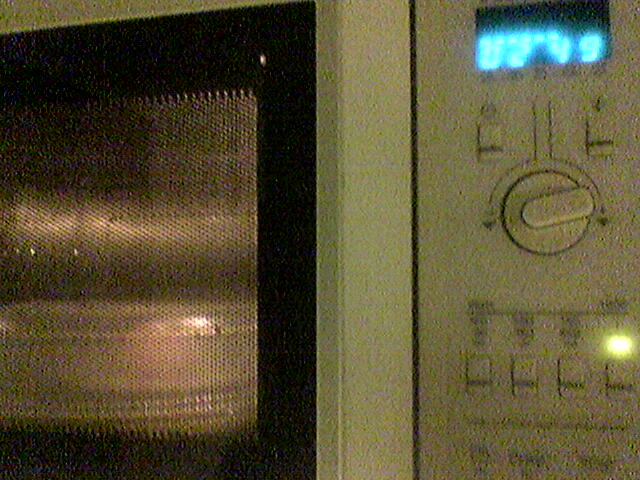This detailed photograph captures a close-up view of an older model white microwave. The image prominently features the control panel on the right-hand side and part of the door on the left. The microwave's door, bordered in black with a semi-transparent, dotted design, reveals a lighted interior with a bowl sitting on the turntable. The control panel includes a black digital display at the top, showing 52 minutes and 49 seconds in white numbers. Directly below the display is a manual timer dial that you turn to set the cooking time, reflecting the microwave's vintage design. Further down, the panel is segmented by a dark brown or gray line, under which three sets of instructions or wording are listed. At the bottom right, there are four square buttons aligned horizontally, each featuring a black line across the center. The rightmost button has a light illuminated above it, adding a functional detail to the scene. The photograph, though somewhat grainy, highlights the nostalgic, knob-and-dial configuration typical of microwaves from several decades ago.